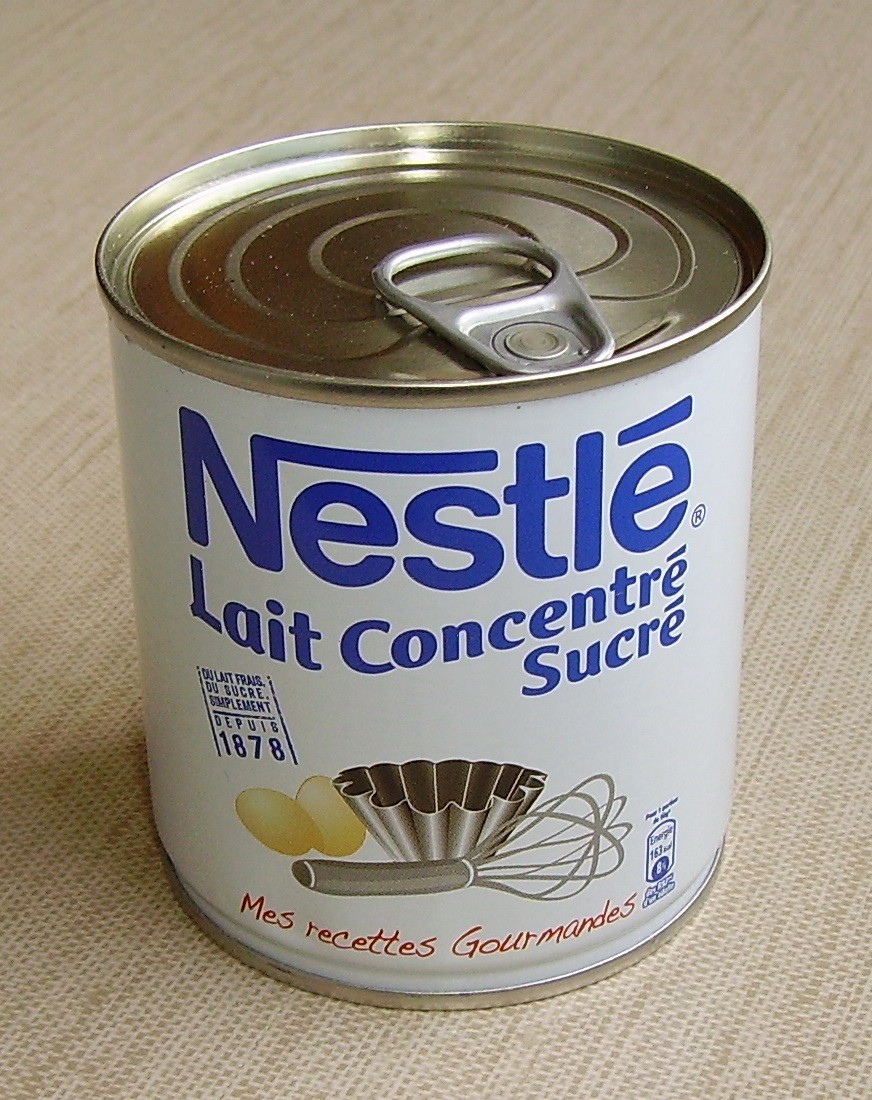This photograph captures a countertop view, taken from slightly above. Prominently featured is a small can with a pull-top lid, adorned with a white label and blue lettering that reads "Nestlé." The remaining text on the label is in a language other than English, adding an international flair. The label also includes a vivid illustration depicting two eggs, a metal basket, and a metal whisk, suggesting the can's contents might be related to baking or cooking. Notably, the label bears the date "1878" on the left side, possibly indicating the year of establishment or a significant milestone for the brand.